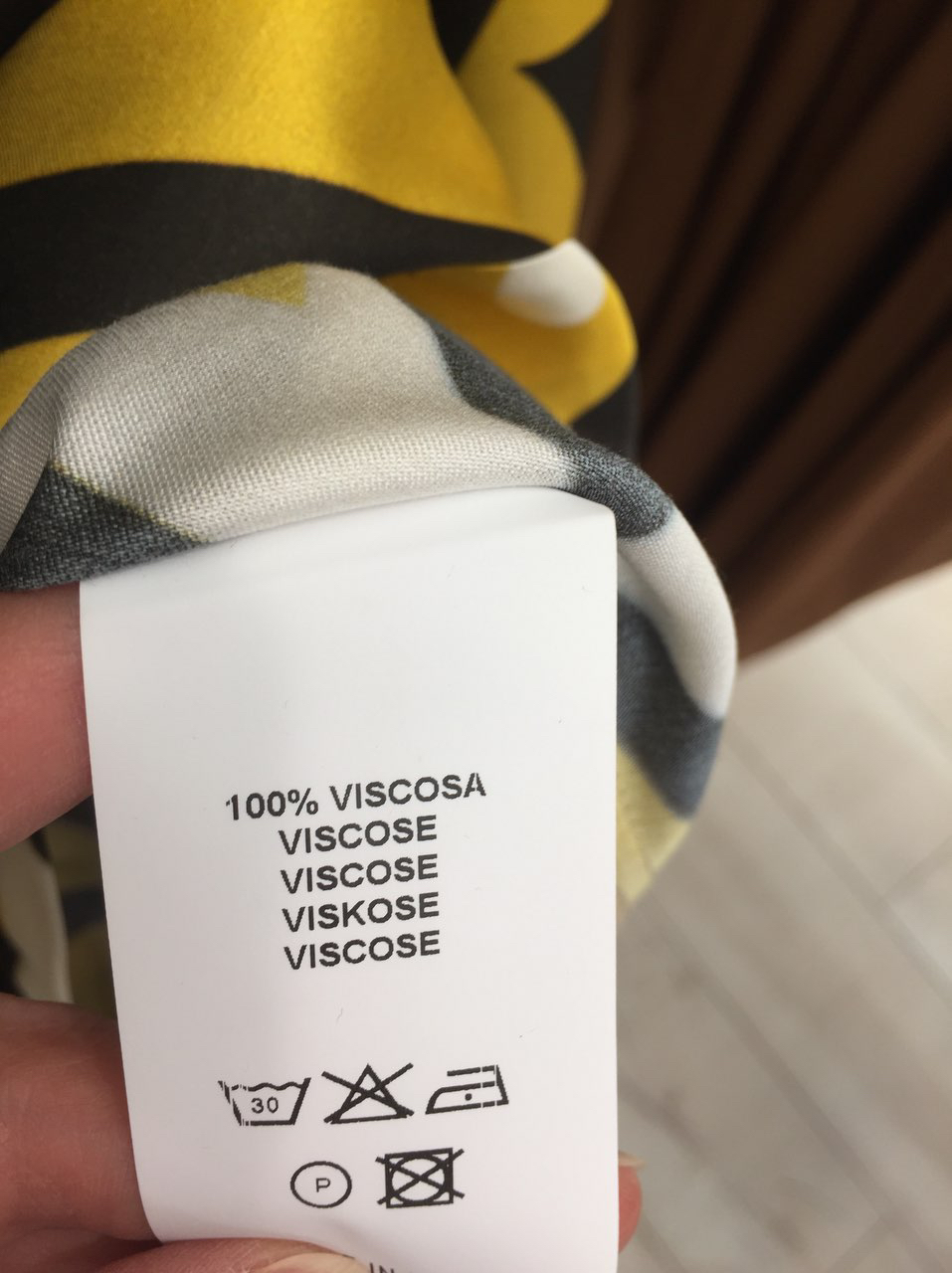The image features a hand at the bottom left, holding a white clothing tag with three fingers—thumb above and two fingers below. The tag is attached to a piece of fabric comprising white, gray, yellow, and black colors, seemingly from a shirt. The background is slightly blurry, showing hints of brown cloth and white wooden planks arranged in thin strips. The white tag displays black text, reading "100% viscosa" at the top, followed by 'viscose' four times, although the third 'viscose' is misspelled with a 'K' as 'V-I-S-K-O-S-E'. Below the text are several laundry care symbols: a cup with '30', a triangle with an 'X', an iron, a circle with 'P', and a square and circle with an 'X'.